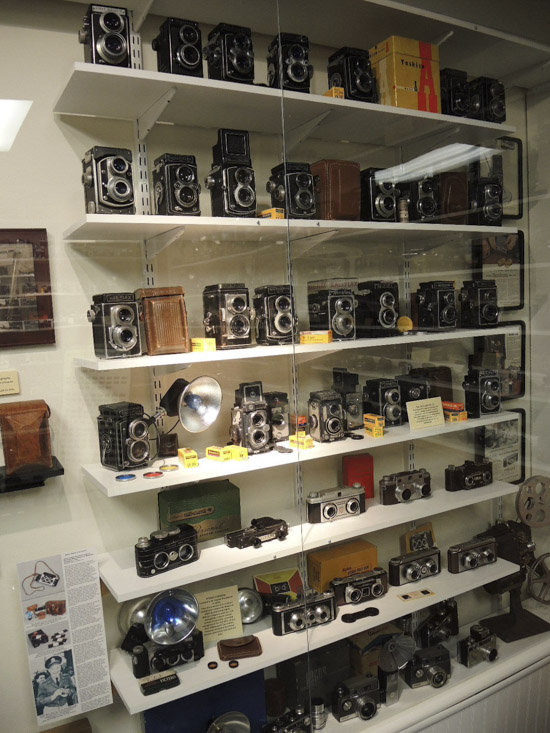The image showcases a glass display cabinet containing an extensive collection of vintage cameras, predominantly characterized by black and silver hues with slight accents of yellow, red, and brown. Displayed on several white shelves, the cameras vary slightly in design but largely consist of dual-lens models, reminiscent of mid-20th-century Leicas. The shelf unit appears slightly tilted towards the right side of the frame, suggesting that the photo was taken from a slight leftward angle. A small, vintage-looking car is also visible on the second lower shelf, adding an eclectic touch to the display. Text is present in the image, though mostly illegible except for a prominently written red "A." The environment resembles a museum or an antique shop, marked by the meticulous arrangement and protective encasement of the cameras, indicating their historical value and aesthetic appeal.